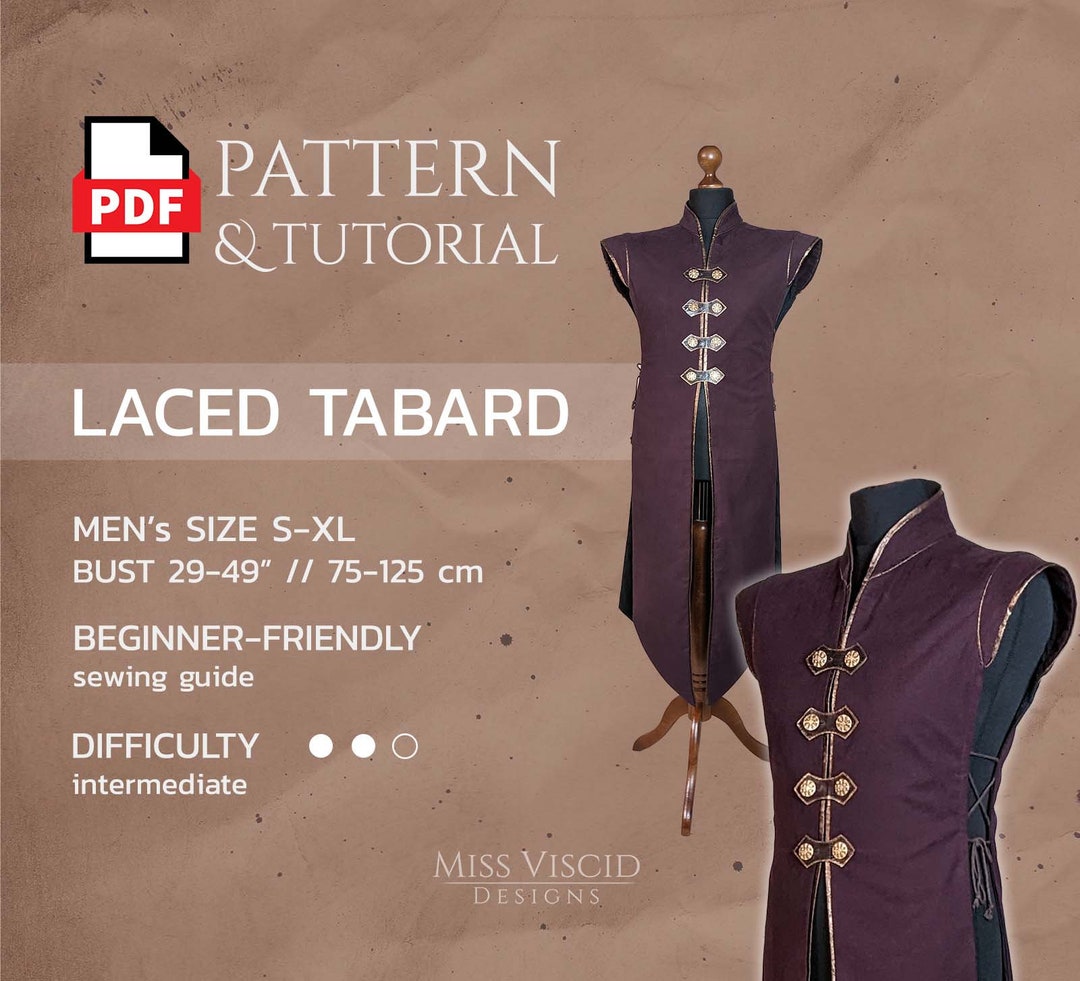This image features a PDF sewing pattern and tutorial for a men's laced tabard, offered by Miss Viscid Designs. The pattern, suitable for men's sizes small to extra-large with bust measurements ranging from 29 to 49 inches (75 to 125 cm), is displayed on a textured tan background. The title "PDF Pattern and Tutorial" is clearly marked at the top in white text on a red background. The laced tabard, shown on headless mannequins, is a tailored sleeveless vest in dark purple and bluish-green hues. It features four tie straps on the chest area, resembling elements of a Chinese uniform or a Nehru jacket. This intermediate-level sewing project, rated 2 out of 3 in difficulty, is designed to be beginner-friendly and is ideal for seamstresses or tailors interested in creating custom garments for men.